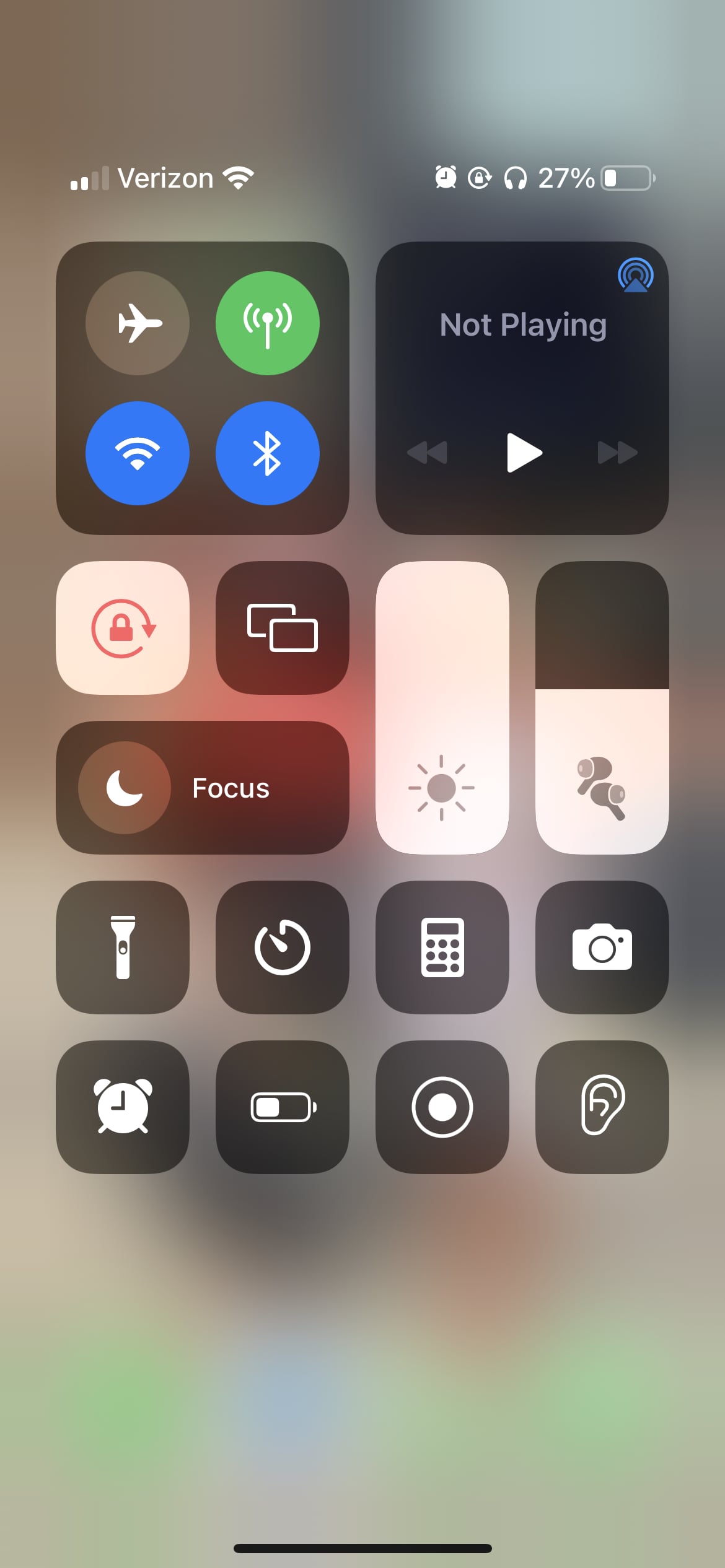The image appears to be a screenshot of an iPhone control center. The background of the image is blurred and filled with various colors like blue, white, green, gray, black, and red. In the top left corner, the status bar is visible showing "Verizon" in white, Wi-Fi signal bars, an alarm clock icon, and a circular arrow icon, all in white. There's also a headphones icon and the battery percentage which reads 27%, both also in white.

The control center consists of several squares and rectangles. At the top, there are two squares with black backgrounds. The first square contains three circles: the leftmost circle is gray with a white airplane icon, indicating Airplane Mode; the middle circle is green and appears to feature a microphone with four lines near it; the last circle under this square is blue and represents the Wi-Fi icon in white. Another icon in this section, consisting of two triangles with two lines, is also present but unrecognizable.

Beneath these icons, there is a music control section with the text "Not Playing" in white. It includes two double-arrow icons on the left and right, and a play button consisting of a white triangle in the middle.

At the bottom of the control center, there are four black squares with white icons indicating a flashlight, time, calculator, and camera. The next row features icons for an alarm clock, battery, a circular symbol within another circle, and something resembling the shape of an ear.

Additionally, there are two squares in the second row: the first is white with a gray sun icon, and the second is half white and half black with gray headphones on the white portion.